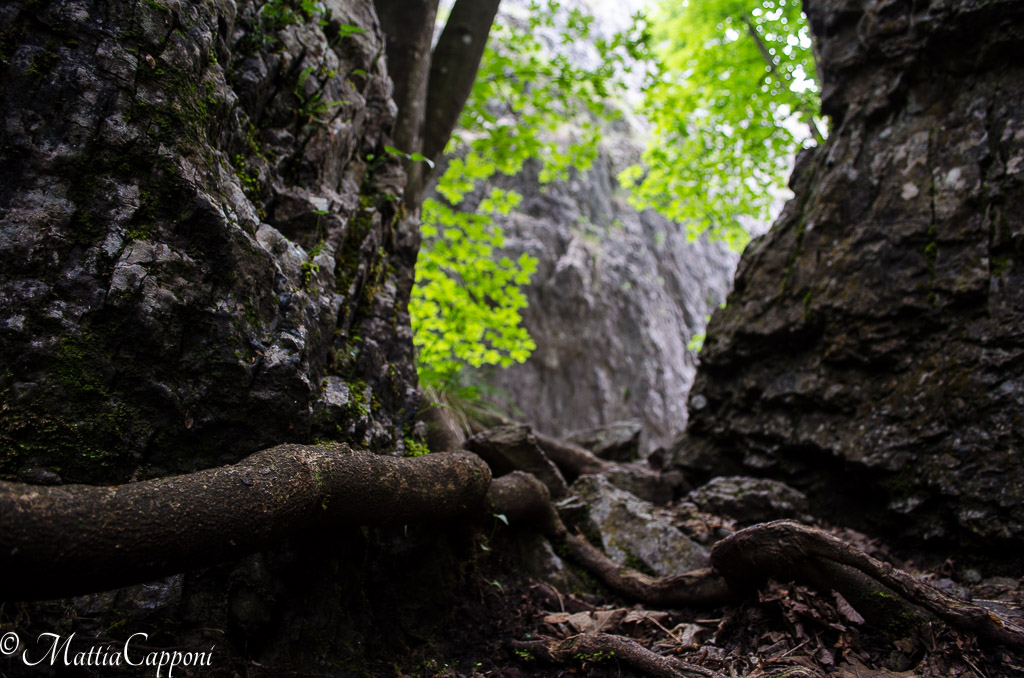The photograph captures the perspective from behind two jagged, large rock faces, revealing a rugged, natural setting. These stone faces, primarily dark green with lighter gray and white patches, flank a gap leading the eyes to another prominent rocky surface in the background. This distant rock face is well-lit and textured, towering vertically with a rough appearance. Between the foreground rocks, a massive tree root stretches across, partially obscured by scattered brown leaves and patches of dirt. Signs of life emerge from the rocks; particularly on the left, where small green leaves and grasses poke through. The scene is bathed in daylight, evidenced by the clear blue sky above and blurry green tree leaves in the distance. The composition evokes a forest ravine or a naturally carved-out area, rich with organic textures and hues. In the bottom left corner of the image, the name "Mattia Caponi" is subtly inscribed.